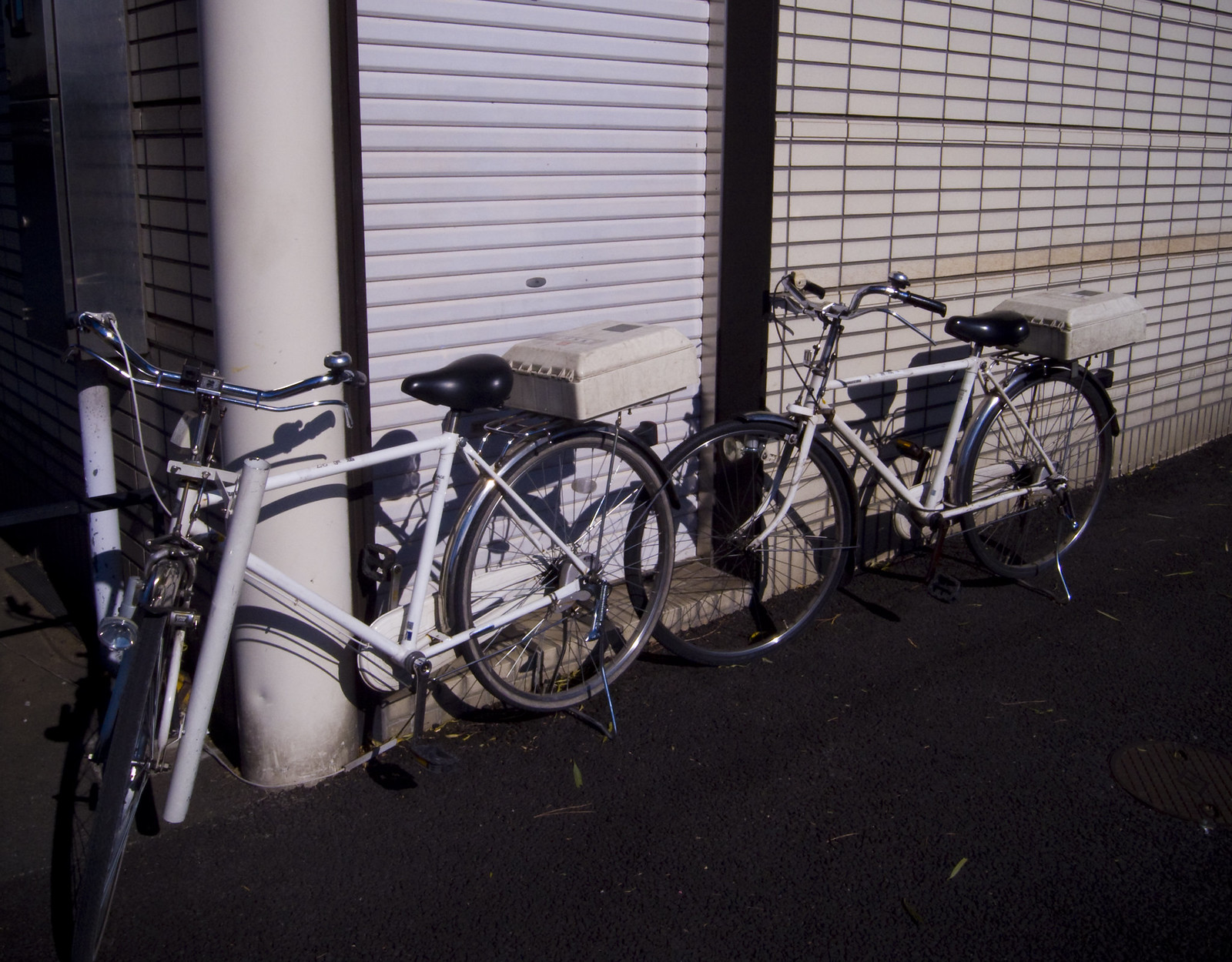In the photograph, two vintage white bicycles with black seats and stainless steel handlebars featuring black grips and bells are parked against a white building. The building has a metal gate and garage-style door, suggesting it might be a closed-down shop. Each bicycle has a white storage pack over the back tire, suitable for carrying items during a ride, and they both rest on their kickstands. The bicycles cast distinct shadows on the building, hinting at the sun beginning to set. The ground in the image is a dark black cement, marked by a manhole cover, contributing to the high-contrast look that makes the scene almost appear monochromatic. The bikes look securely locked to the building or posts, emphasizing their unattended yet secure position.